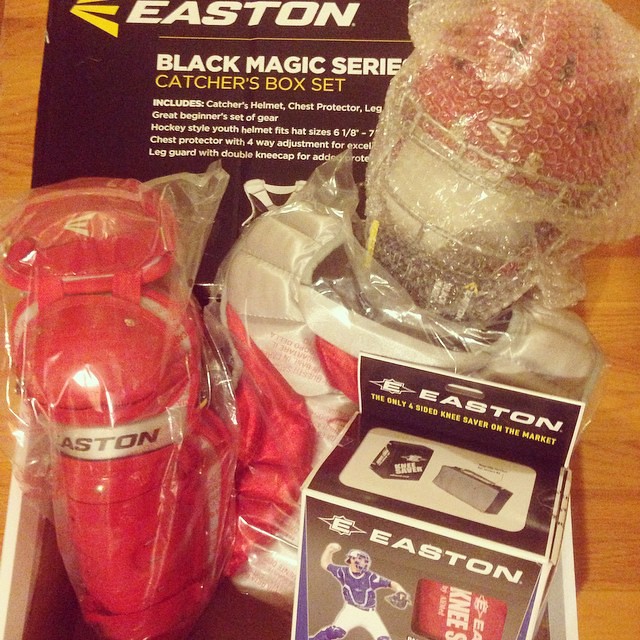In the image, a detailed unboxing of Easton sports gear is displayed on a medium brown wooden counter with darker grains. The background features a black box with the Easton logo in large white letters, followed by "Black Magic Series" also in white, and "Catcher's Box Set" in yellow. Below, white text lists included items: a catcher's helmet, chest protector, leg guards, and more, though some text is obscured by the gear. The box also mentions, "Great beginner's set of gear," "Hockey style youth helmet fits hat size 6 1/8 to 7...," "Chest protector with 4-way adjustment for XL fit," and "Leg guard with double knee cap for additional protection," though some of this information is partially cut off.

Prominently displayed in the center of the image, surrounded by plastic wrap and bubble wrap, are three main items: on the left, a red piece of gear labeled Easton, likely a protective cup; in the middle, gear intended for knee protection also bearing the Easton logo; and in the top right, a red helmet with ventilation holes, wrapped in bubble wrap. At the bottom right, another package is visible, marked with the Easton logo, stating "The only four-sided knee saver on the market." Additionally, part of a box with an image of a baseball player and possibly a close-up of a knee guard is visible, further emphasizing the comprehensive nature of the catcher's set.